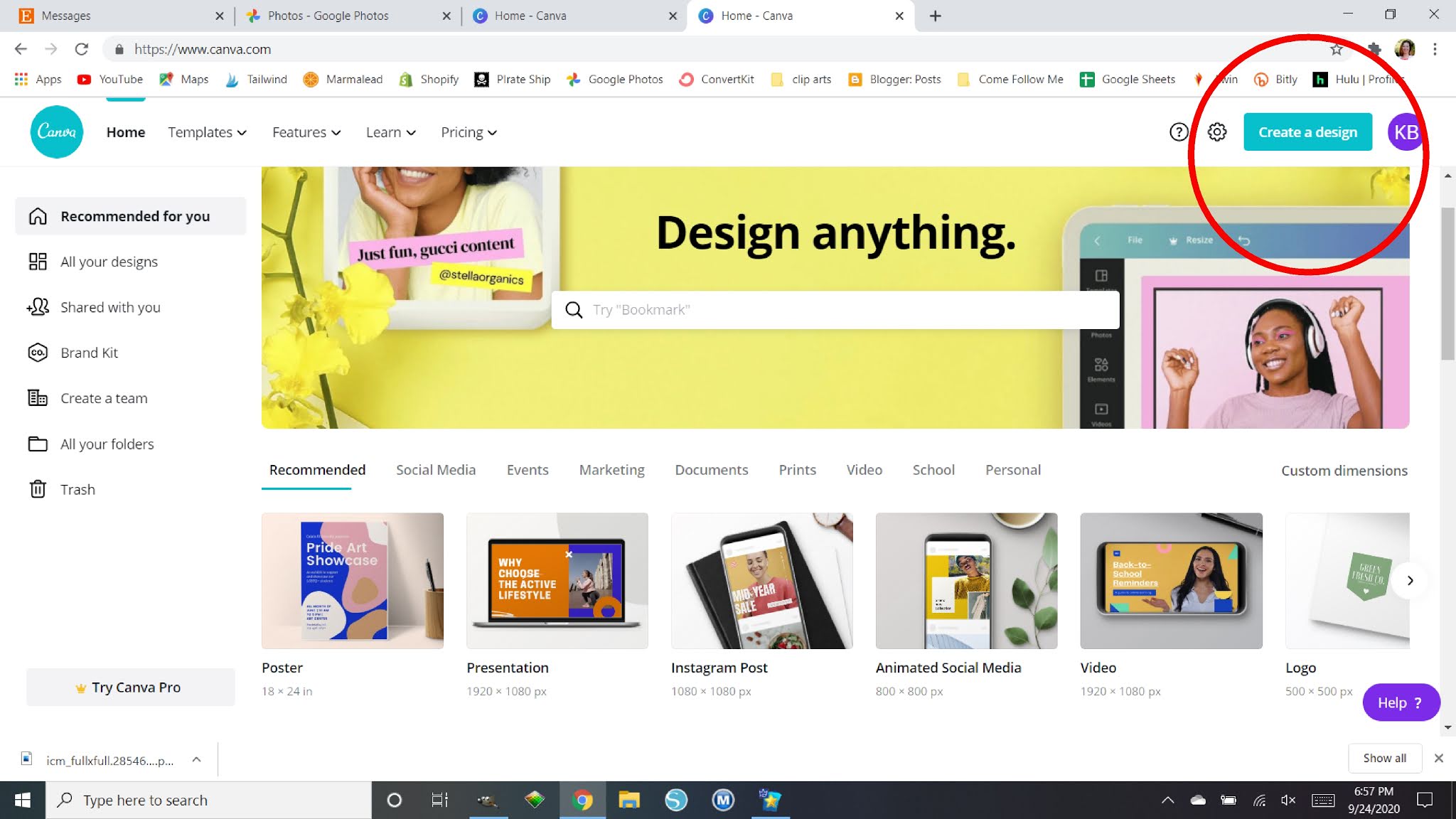The image depicts a computer screen displaying a web browser with multiple tabs open. At the top, the tabs include "Messages," "Photos - Google Photos," "Home - Canva," a duplicate "Home - Canva," each marked with an 'X' for closing. Additionally, there is a prominent black plus sign symbolizing an option to open a new tab. To the right of this plus sign, there's an icon featuring a minus sign inside a square, followed by another 'X'.

In the main browser window, the search bar displays the URL "https://www.canva.com." Below this, various app icons are listed, including YouTube, Maps, Tailwind, Marmalade, Shopify, Pirate Ship, Google Photos, ConvertKit, Clip or Blog Post, "Come Follow Me," Google Sheets, Bitly, Hulu, "Profile," "Create a Design," and a user-named "KB," which is encircled in red.

To the left, a sidebar menu features options such as "Recommended for You," "All of Your Designs," "Shared With You," "Brand Kit," "Create a Team," "All of Your Folders," "Trash," and an option to "Try Canva Pro" marked with a crown icon. At the bottom, a file appears to be in the process of downloading. Finally, beneath the main content, another search bar is present, showing the Google symbol and an "M" within a circle.